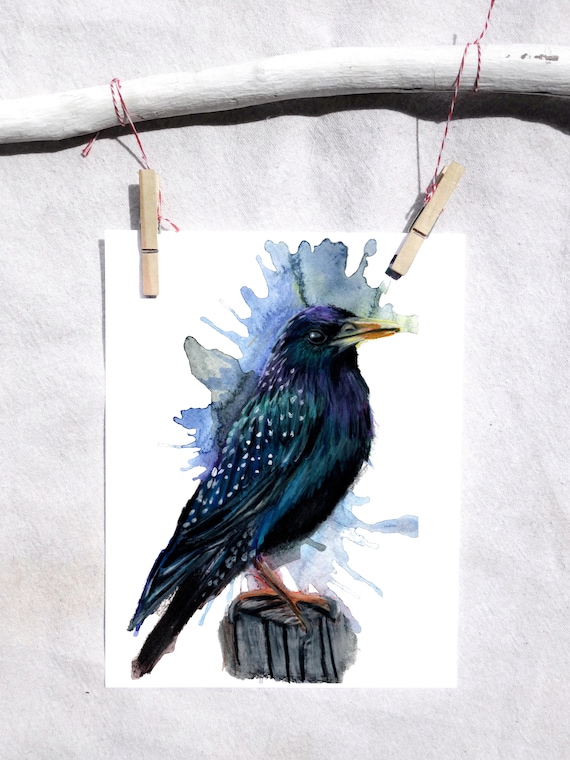This detailed image, captured in a photograph, showcases a striking painting suspended by two wooden clothespins. The painting hangs from thin red and white string tied to a sun-bleached, whitewashed branch, which rests on a backdrop of white sand. The artwork itself features a black bird, likely a crow, with iridescent white spots on its feathers that reflect hints of blue, green, and even a touch of purple. This avian subject stands on a piece of worn, reclaimed wood, and is set against a white background that is accentuated by a vivid blue watercolor splotch, giving the impression of paint spreading like on a soaked paper towel. The bird’s beak and feet are a striking gold color, adding vibrancy to the scene. The combination of elements – the whitewashed branch, the clothespins, the string, and the bird’s colorful detail – culminates in a visually captivating composition.